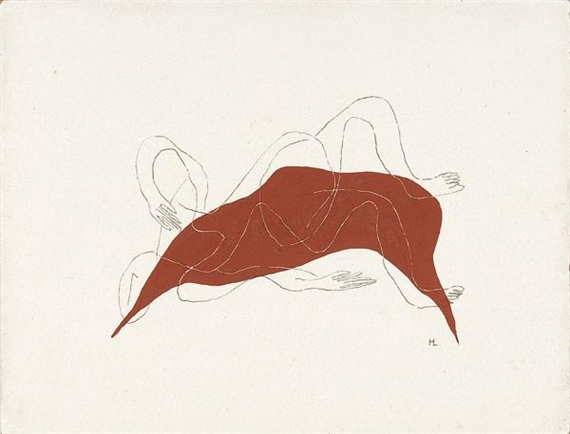The image features an intricate abstract composition set against a stark white background. Dominating the center is a central, reddish-brown shape reminiscent of a scarf or a leaf, curving gracefully from left to right with pointed ends. Surrounding this central figure is a wavy, fluid outline that resembles the form of a person, complete with abstract arms and legs extending from the central shape. The arms curve naturally with discernible fingers, and the legs, emerging from the central mass, arc gracefully, contributing to the overall fluidity of the piece. Above and below this central shape, thin, sketch-like white lines loop around in circular patterns, further enhancing the abstract nature of the artwork. At the bottom right corner, there's a partially legible artist's signature, possibly starting with an "H" or "M."